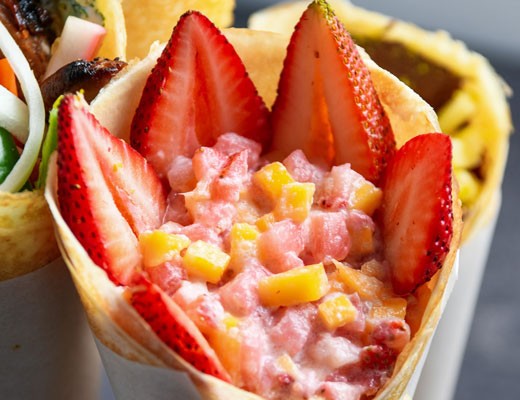The image showcases a variety of crepes, prominently featuring a visually appealing breakfast bowl style crepe. The main crepe is artfully arranged with six sliced strawberries lining the inner edge of a funnel-shaped or shell-like wrap, which appears to be made of a crepe or pancake. In the center of the strawberry-lined crepe, there is a colorful mixture of chopped fruit pieces and a pinkish sauce or mass. To the upper left, the image partially captures another savory crepe filled with what seems to be meat, onions, and bell peppers. In the background, there are glimpses of additional crepes wrapped in white paper, each containing different, indistinguishable fillings. The composition of the image highlights both the sweet and savory aspects of these delicious-looking crepes.